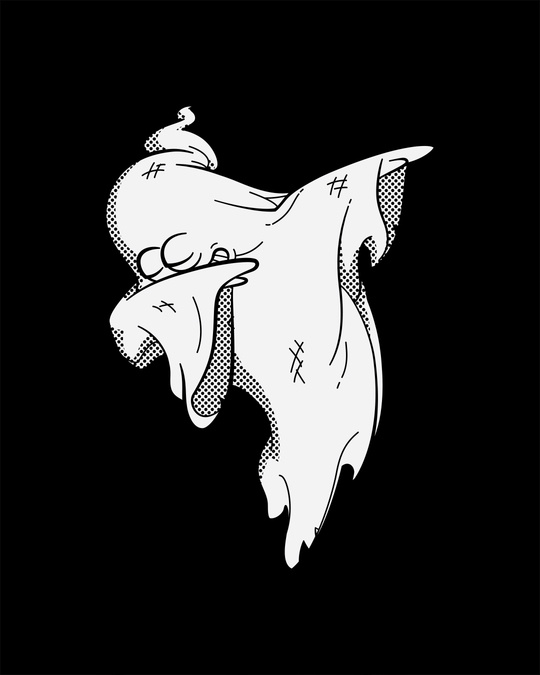The image is a black and white, cartoon-style illustration set against a solid black background. In the center of the portrait-oriented frame is a simple yet expressive white ghost, appearing to float. The ghost is depicted in a 'dabbing' pose, with one arm crooked and covering its face while the other arm extends outward. Its head tilts downward, and it has its eyes closed, suggesting a sense of concentration or playfulness. A small curlicue adorns the top of its head, reminiscent of a swirl of ice cream. The inside of the ghost's robe features black-and-white checkered patterns, while the overall garment is slightly worn, indicated by random black hash marks and scuffed edges. The character’s endearing grin is subtly visible at the side of its mouth. The ghost’s two visible fingers and oddly shaped, curved lower edges contribute to its whimsical, cartoony design.